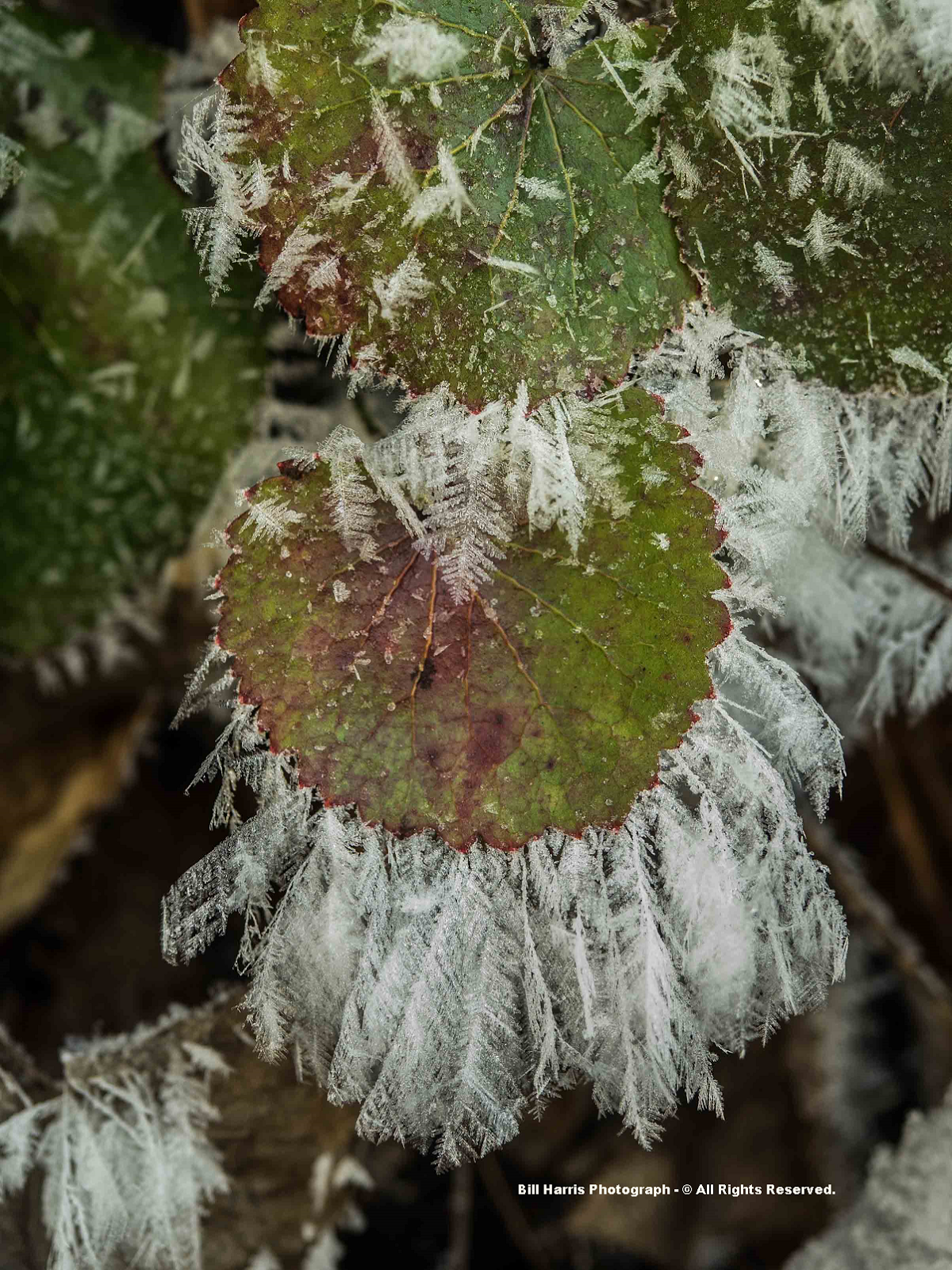The image depicts a plant that appears to belong to the succulent family. The plant features green leaves with rust-colored discolorations at their centers. The leaves are adorned with clusters of fine, thin, spiky white outgrowths that resemble feathers or seeds, suggesting the plant may be in a stage of pollination or germination. There are approximately two to four prominently visible leaves in the foreground, each displaying these characteristic features. Below the plant, a word is written, and the background includes blurry sections on the left side and the bottom right side of the image.